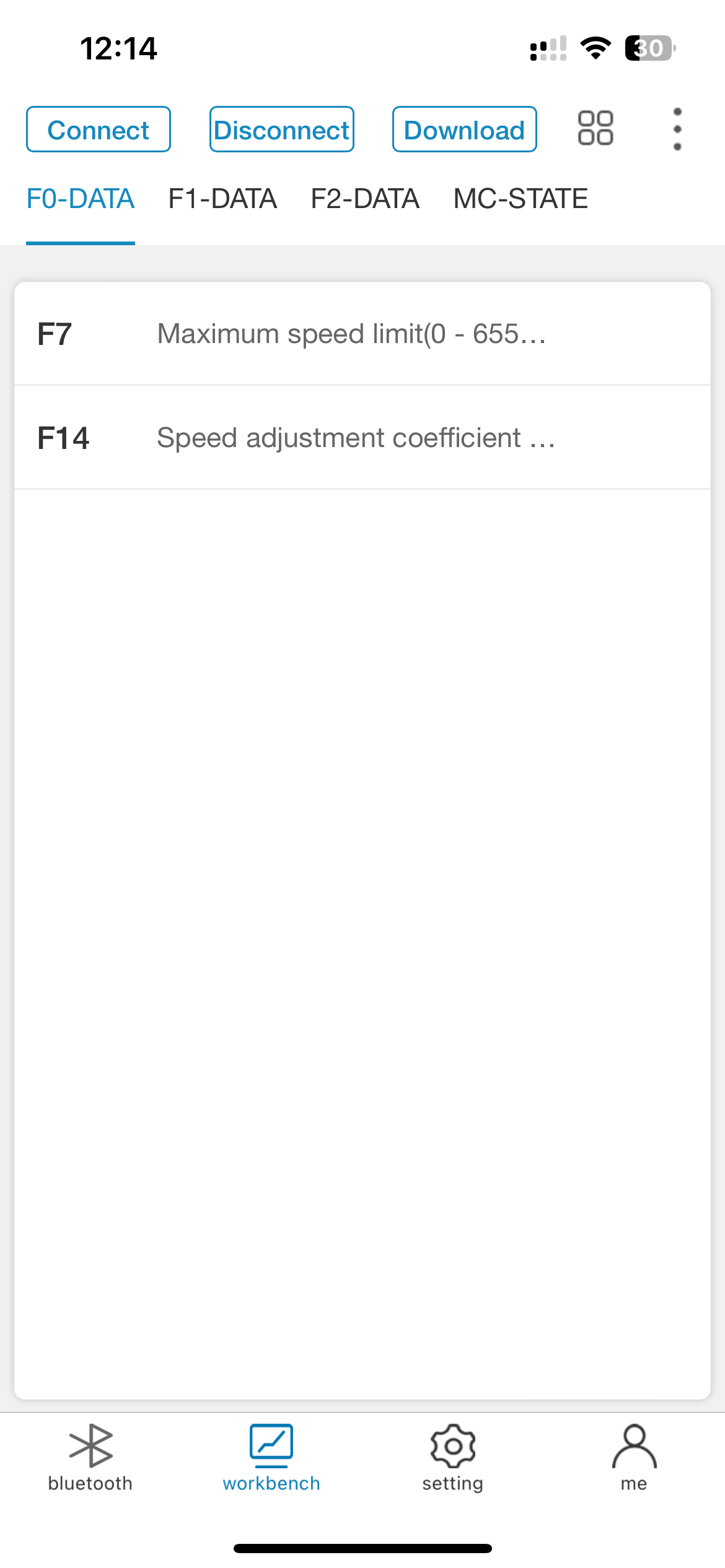**Detailed Caption:**

The image is a screenshot of a smartphone's screen, displayed on a white sheet of paper. The screenshot predominantly has a white background. At the very top, the status bar shows a network signal strength of less than two bars, the time displays as "2:14," and the battery life is indicated at 30%.

Beneath the status bar, there are three rectangular buttons aligned horizontally. Each button has a white interior with a blue border and blue text. From left to right, the buttons are labeled "Connect," "Disconnect," and "Download." To the immediate right of these buttons, there are four small squares arranged in a 2x2 grid, which likely represent a thumbnail or grid view option. Further to the right, three vertical dots suggest an expandable menu.

Below this horizontal menu, there is a row of options written in blue text with underlines, indicating clickable links. These are labeled from left to right as "FO data," "F1 data," "F2 data," and "MC state."

In the main screen area, at the top, bold black text displays "FS." To the left of "FS," in gray text, it reads "Maximum speed limit, 655." Below this, another line in bold text says "F14," with "Speed adjustment coefficient" written underneath in smaller text. This is the entirety of the visible information on the screen.